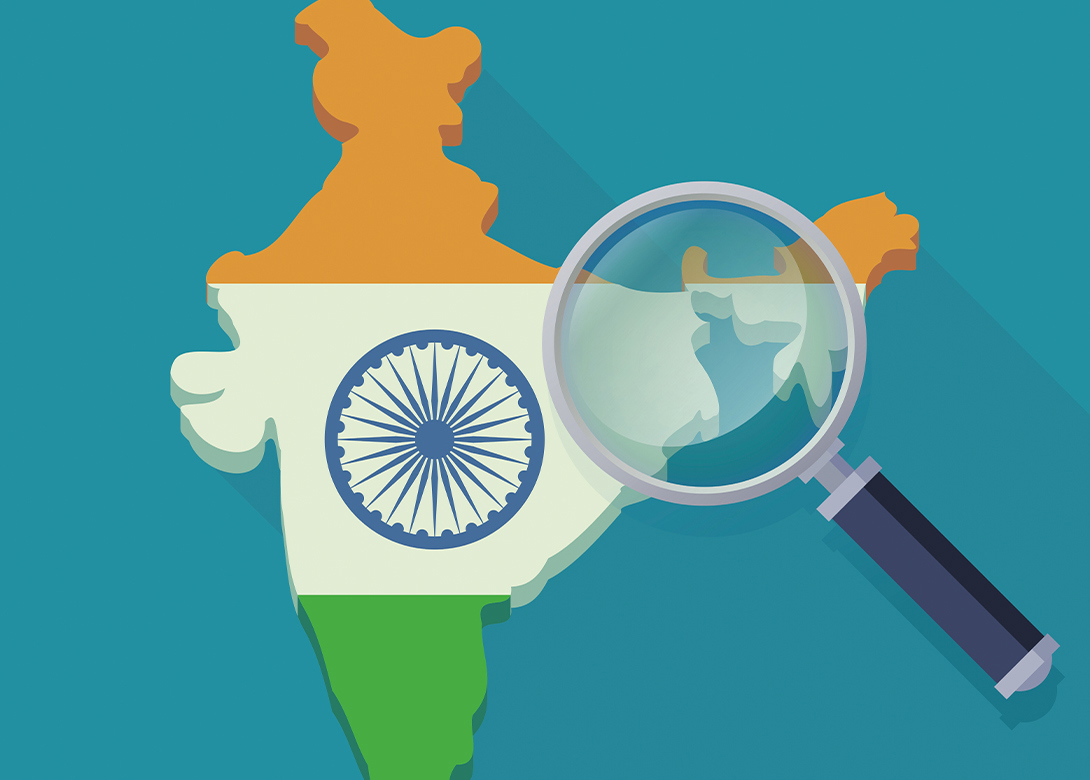The image features a solid, dull blue background upon which a color-divided, three-dimensional map outline is displayed. This map, resembling the shape of a country, is divided into three distinct horizontal sections: the top part is yellowish-orange, the middle part is white featuring a blue circle with spiky protrusions, and the bottom part is light green. The map itself suggests the form of a country or region, with a skinny top portion that widens in the middle before tapering off again at the bottom. Positioned prominently over this map is a magnifying glass, emphasizing the blue circle and its surrounding spikes. This magnified segment sits within the white middle section of the map. The map's design hints at a flag, as the three colors are arranged in horizontal bands. The overall setting, along with the magnifying glass, suggests an analytical or exploratory theme.